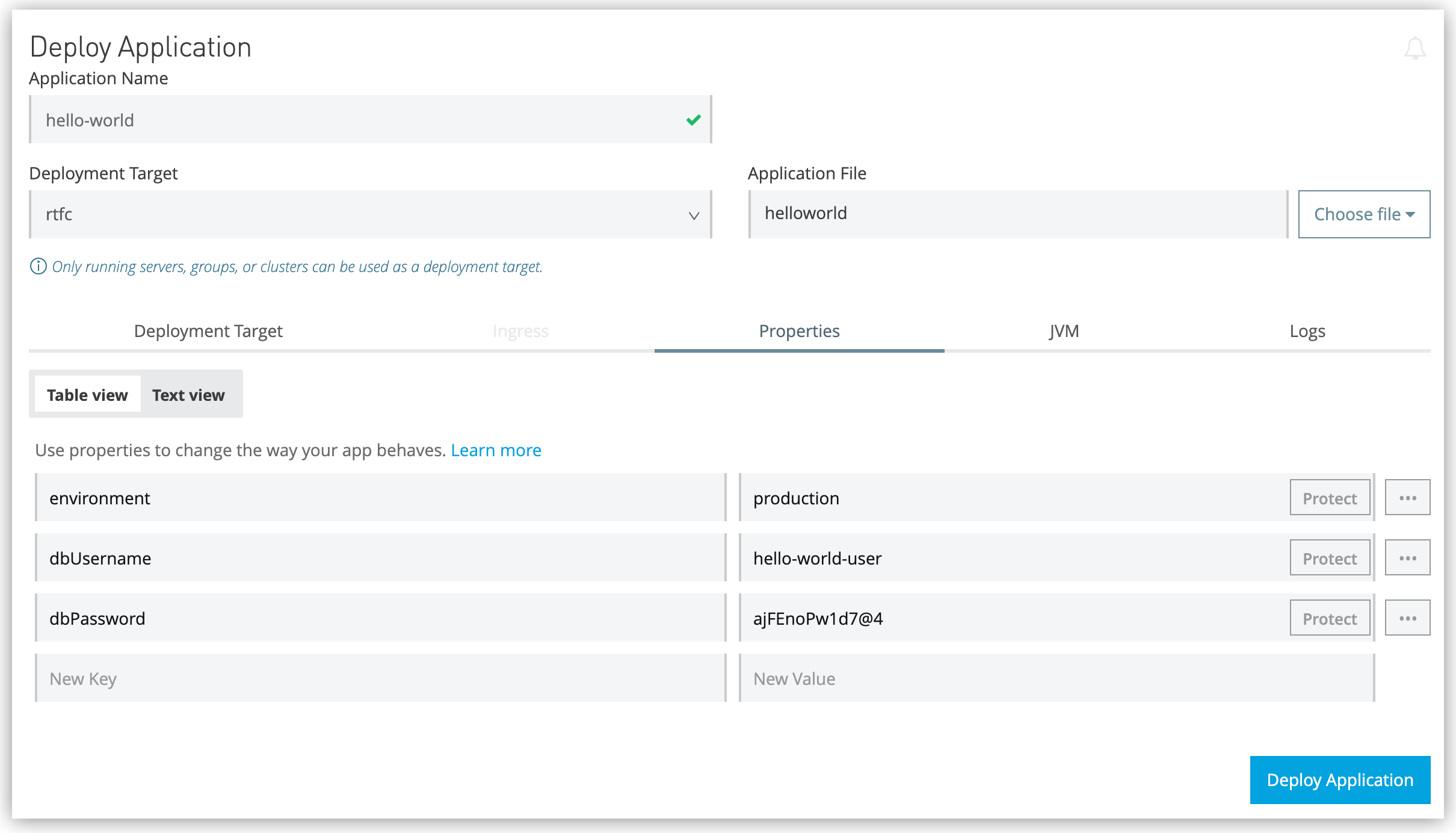The image depicts a deployment page for an application with mainly white and light gray backgrounds. At the top of the page, there is a section where the application name is displayed as "hello-world." The deployment target is set to "rtfc," which is chosen from a dropdown menu. A nearby information icon indicates that only running servers, groups, or clusters can be used as deployment targets. The application file, named "hello-world" without spaces or dashes, is also specified, and there is an option to choose a different file.

Further down the page, in the properties subsection, users can configure various settings to alter how the application behaves. These properties include variables like "environment," "DB username," and "DB password," which likely pertain to database configurations, enabling the application to access necessary information. At the bottom right of the page, there's a prominent "Deploy Application" button, signifying the final step in initiating the deployment process.